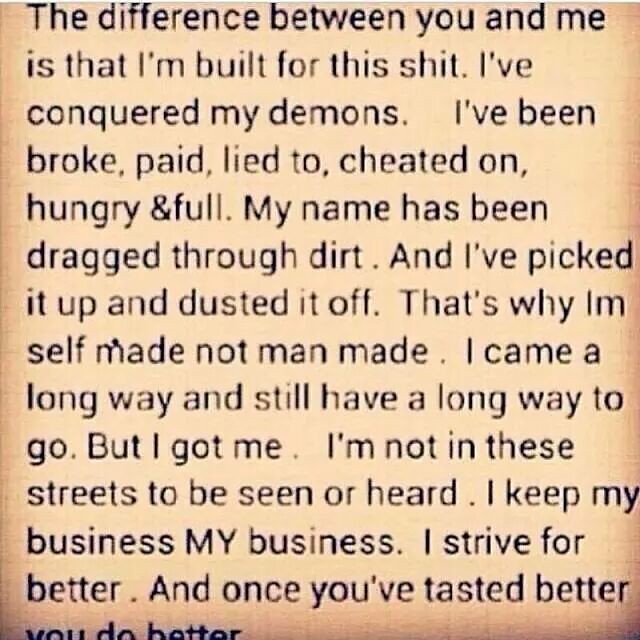The image depicts a text written in aged black font on a beige piece of paper that gives it an old, worn appearance. The words span the length of the paper from top to bottom and read: "The difference between you and me is that I am built for this shit. I've conquered my demons. I've been broke, paid, lied to, cheated on, hungry and full. My name has been dragged through dirt, and I've picked it up and dusted it off. That's why I'm self-made, not man-made. I came a long way and still have a long way to go, but I got me. I'm not in these streets to be seen or heard. I keep my business my business. I strive for better, and once you've tasted better, you do better." The background suggests the text might be from a book or possibly posted on a website, adding to its reflective and motivational essence.